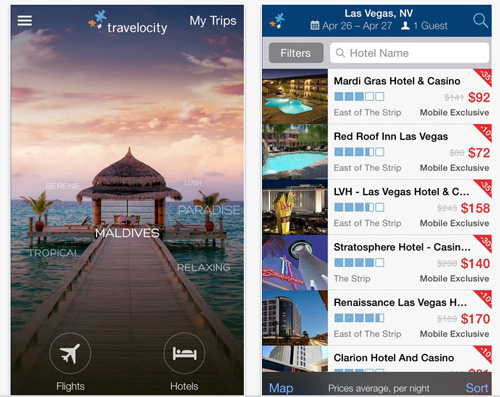The image is divided into two sections showcasing the Travelocity app interface. The first section features the Travelocity app icon, which is small and colored in a blend of blue, orange, and green, with "Travelocity" written in white text alongside the "MyTrips" label. Accompanying this is a picturesque beach scene that invites a stroll right to the water's edge, with overlay text highlighting destination keywords such as "Tropical," "Maldives," "Relaxing," and "Paradise." Prominent white icons for flight and hotel, each represented with an airplane and a bed respectively, are also displayed.

The second section presents a detailed search result for hotels in Las Vegas, Nevada, for a stay from April 26th to 27th for one guest. It includes several filters and features listings such as:

- **Mardi Gras Hotel and Casino**: Located east of the Strip, featuring an image of a pool and hotel, priced at $92, marked down by 35% from the original $141, and noted as a mobile exclusive.
- **Red Roof Inn Las Vegas**: Also east of the Strip, featuring a pool, priced at $72, marked as a mobile exclusive.
- **LVH Las Vegas Hotel and Casino**: Located east of the Strip, priced at $158, noted as a mobile exclusive.
- **Stratosphere Hotel and Casino**: Situated on the Strip, priced at $140.
- **Renaissance Las Vegas**: East of the Strip, priced at $170.

Most of the text on this page is in black, with prices and discount percentages highlighted in red, emphasizing the savings available.